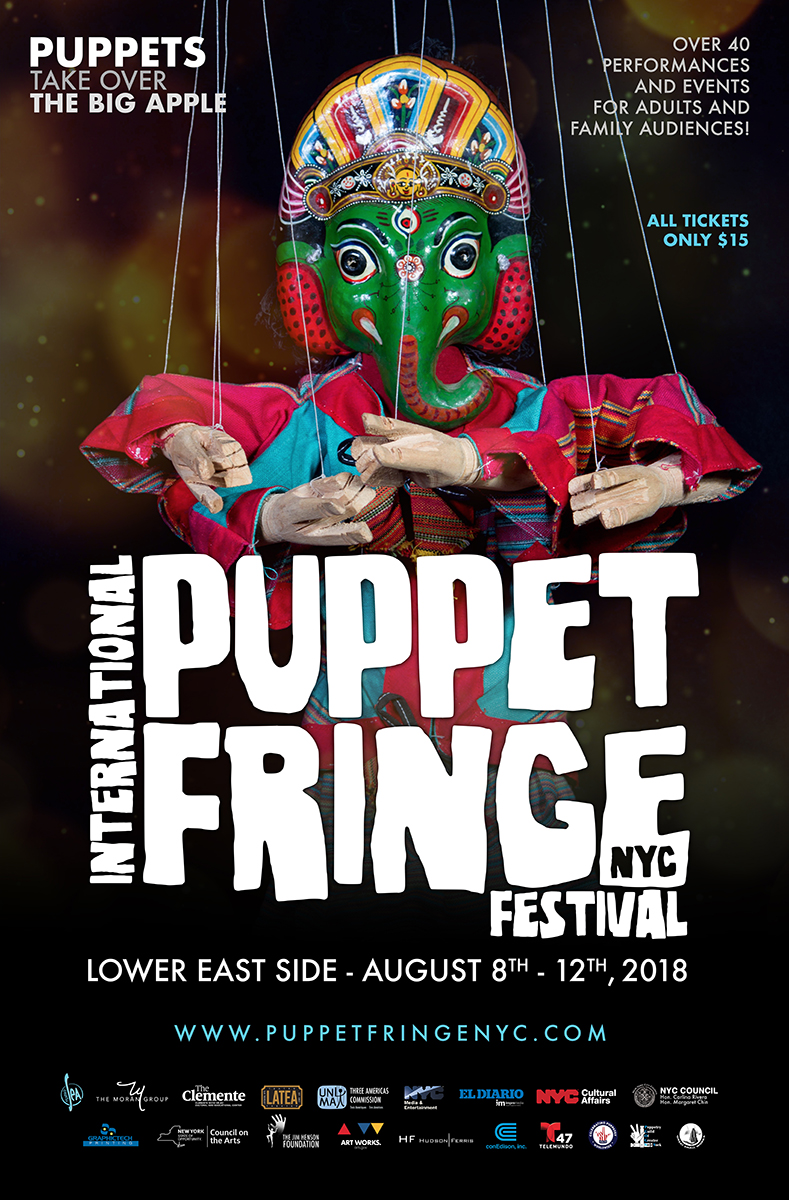This promotional poster advertises the International Puppet Fringe Festival in New York City, held on the Lower East Side from August 8th to 12th, 2018. The poster features a striking black background with a prominent image of a complex puppet that resembles an Indian god, complete with an elephant face and four arms, hanging from strings. Key details include the event’s slogan, "Puppets Take Over the Big Apple," and information about over 40 performances and events suitable for both adults and families. An eye-catching detail is the blue text in the upper right corner stating, "All tickets only $15." The poster also highlights the festival's website, www.puppetfringenewyorkcity.com, with NYC abbreviated, and a series of sponsor logos running along the bottom border.